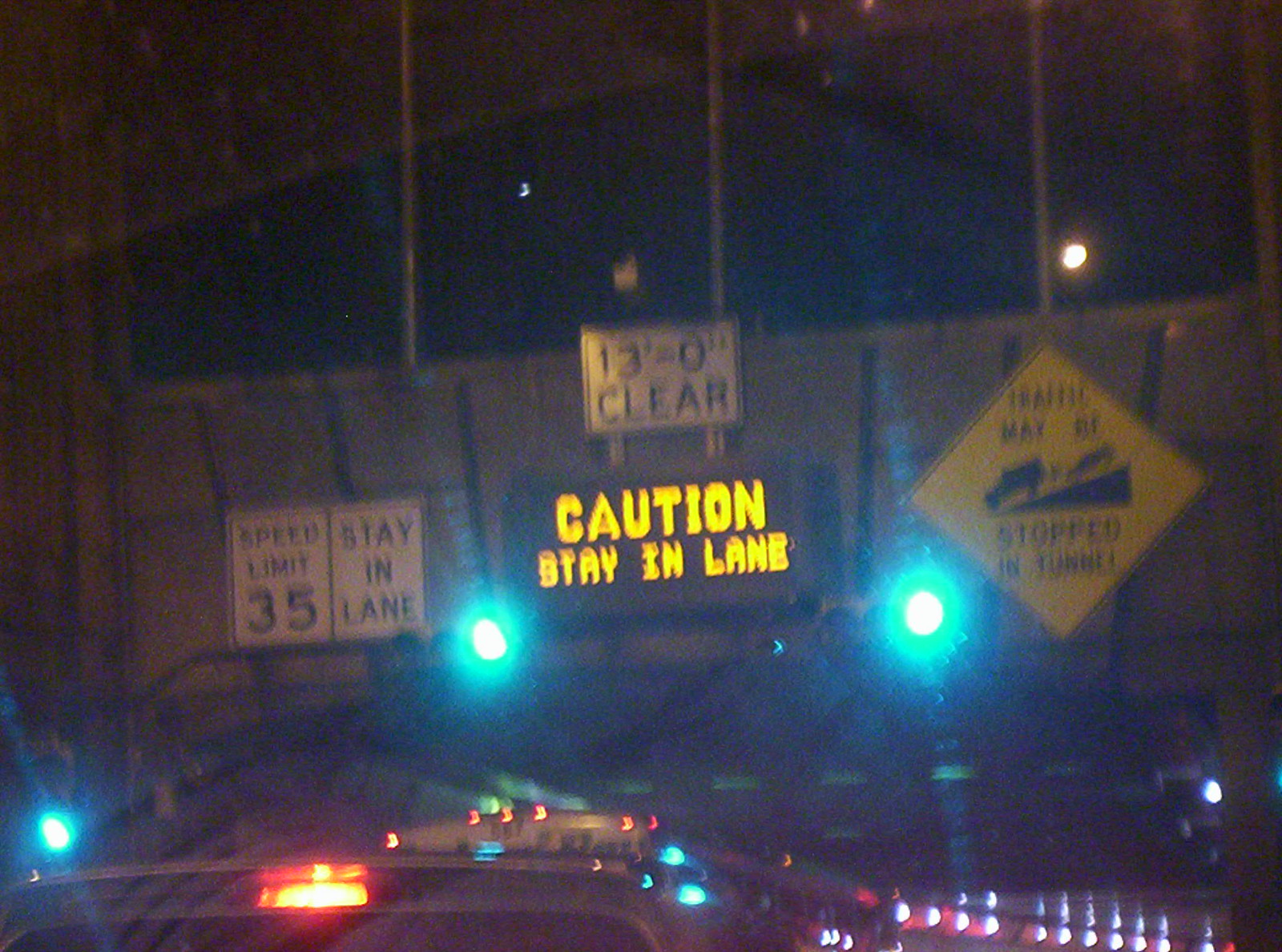This is a blurry, low-quality photo taken at night, presumably from a car stuck in traffic at the entrance of a tunnel. The image, captured through a windshield, shows several vehicles with their lights on, though they are hard to make out clearly. Dominating the scene is a large bridge-like structure with various signs. To the left, there's a white sign with black lettering indicating a speed limit of 35 mph and a matching sign next to it reading "Stay in Lane." In the center, a yellow and black electronic sign displays "Caution Stay in Lane," situated below another sign stating "13 Feet 0 Inches Clearance." On the right, a yellow diamond-shaped sign warns that "Traffic May Be Stopped in Tunnel" with an icon of a truck. The entrance is adorned with several blue and white lights along the base, and you can also see structural posts descending from the top. This disorganized array of traffic control signs and lights suggests an area under careful regulation as vehicles queue to enter the tunnel.